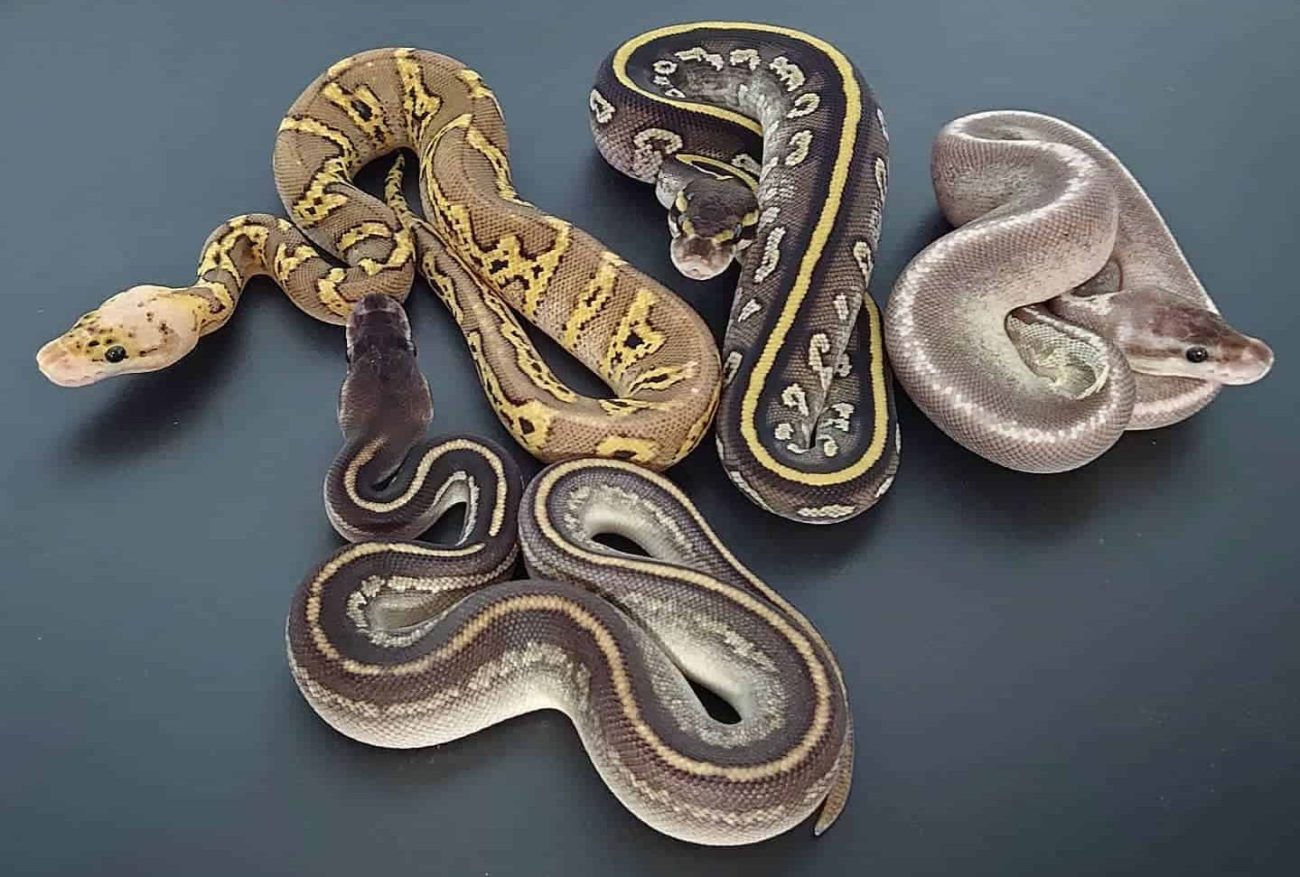This is an image of four snakes resting on a dark teal-blue surface, with a slightly angled perspective that shows them in different curled configurations. In the foreground, a snake with black and white coloring and a light brown stripe down its back faces the ones behind it. Its head is lifted, poised attentively at another snake. To the left in the background, a light brown snake with golden splotches and a peach-colored head looks off to the left with its head raised. The middle snake in the background is dark with white patterns and features a yellow stripe down its back, and it is staring directly at the camera. The snake on the right has a shiny, almost metallic silver color with a distinctive stripe along its back, looking off to the right with its head resting on its coiled body. The entire scene presents a diverse array of snake varieties against the dark backdrop, with subtle details in their patterns and poses.